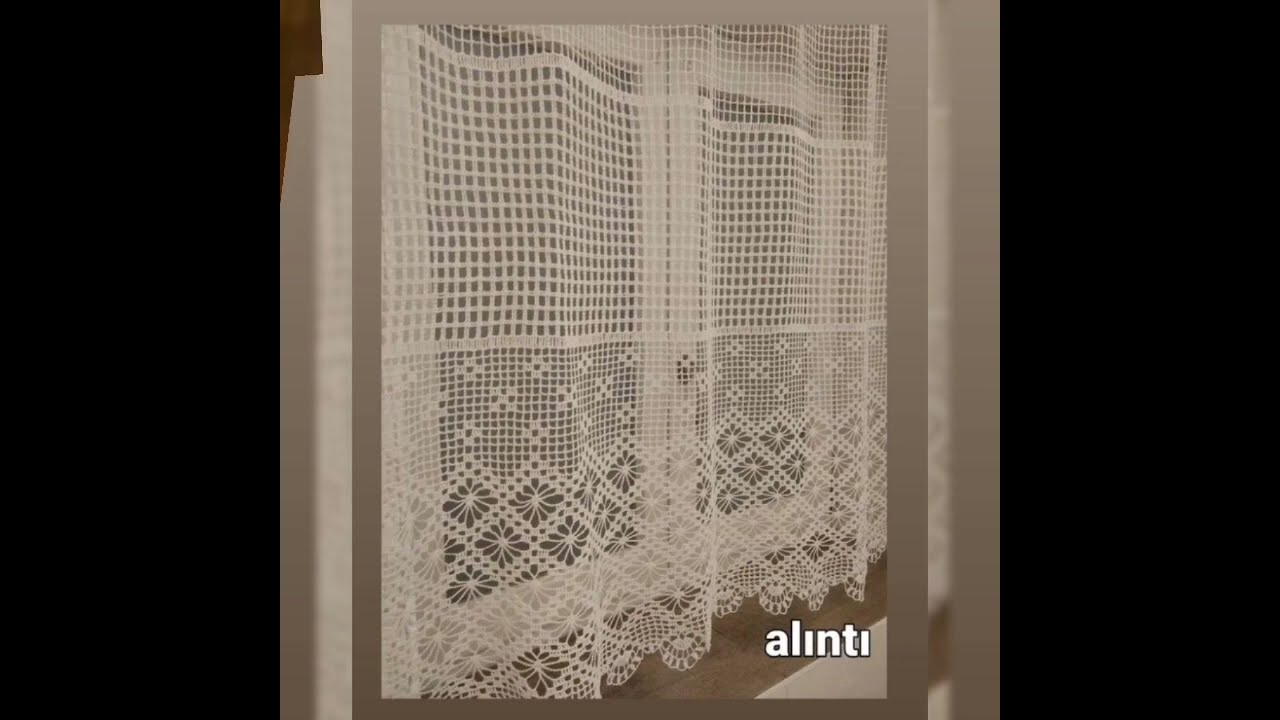This indoor photograph presents a predominantly white scene centered around a semi-transparent, decorative curtain made of white, lacy material. The curtain, featuring various intricate patterns including small squares at the top and diamond shapes at the bottom, hangs centrally from top to bottom against what appears to be a door or window. The door or window behind the curtain includes a small latch in the middle, partially obscured by the fabric. Framing the curtain are vertical black rectangular spaces on either side, which might be part of the photograph's border. The composition is primarily white with hints of gray and off-white, lending a serene and minimalistic feel. In the bottom right corner of the photograph, the word "alinti" is discreetly printed in lowercase.